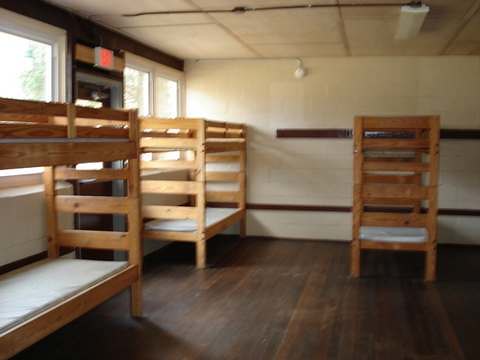The image depicts a sparsely furnished room, potentially a barracks or dormitory, characterized by its stark simplicity and utilitarian design. The room features three wooden bunk beds with very thin, white mattresses, devoid of any bedding or pillows. These bunk beds, made from light to medium brown timber, are arranged with two on the left side of the room and one on the right side. 

The left side of the room houses two windows, which flank a dark brown emergency exit door marked by a glowing red exit sign above it. The windows offer a blurred view of green foliage, indicating the presence of trees outside. Both walls and ceiling are stark white, with the walls constructed from painted concrete blocks. Horizontal strips of dark-stained wood decorate the upper half of the walls, adding a sparse decorative element.

The room's flooring is dark wood, contrasting sharply with the white walls. The ceiling is a drop-down style, fitted with large fluorescent light fixtures, adding to the room's functional and austere ambiance. The overall layout and features, such as the basic lighting and emergency signage, suggest a practical space designed for temporary accommodation, emphasizing utility over comfort.